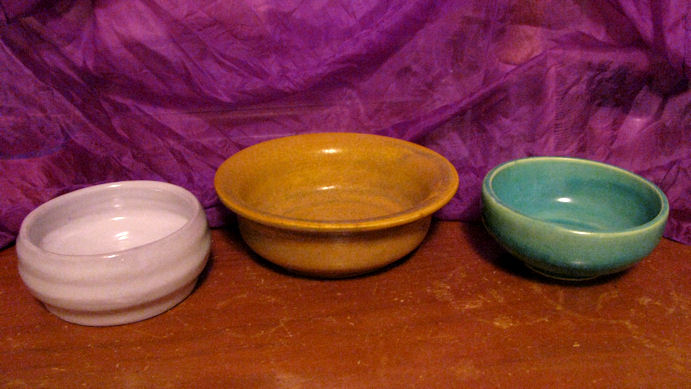Three hand-cast and hand-glazed ceramic bowls are arranged on a well-worn and scratched wooden table, visible from a slightly overhead perspective. Each bowl is uniquely shaped and colored: the first is an earthy pink with a tiered design, the second is an earthy ochre with a notably wide lip and is the largest of the three, and the third is a green bowl that transitions from light green at the top to a darker green mixed with brown at the base. The wooden table has signs of extensive use, including moisture rings and a stick figure scratched into its surface. In the background, a wrinkled and faded purple cloth, almost maroon in places, hangs, adding texture to the scene. The photograph appears to be set up for advertising the handcrafted quality of these distinct bowls.